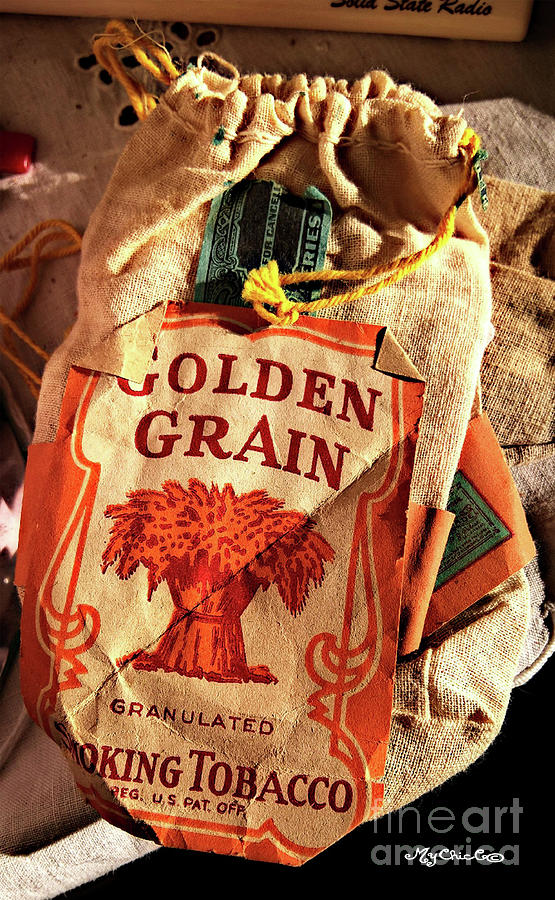This detailed photograph captures an empty canvas sack with yellow drawstrings labeled "Golden Grain" and adorned with an image of bundled wheat. Beneath this, the label reads "Granulated Smoking Tobacco Reg. U.S. Pat. OFF." The sack is prominently featured and rests on top of a stack of identical sacks. The perspective of the shot is from above, looking down at the sacks, revealing a workshop-like background with a wooden floor. The bottom right corner displays the Fine Art America copyright and "My Circle" logo, emphasizing the image's ownership. The top of the sack has some indistinct writing with the partially visible word "radio." The bottom portion of the photograph is darkened, further highlighting the Fine Art America copyright.